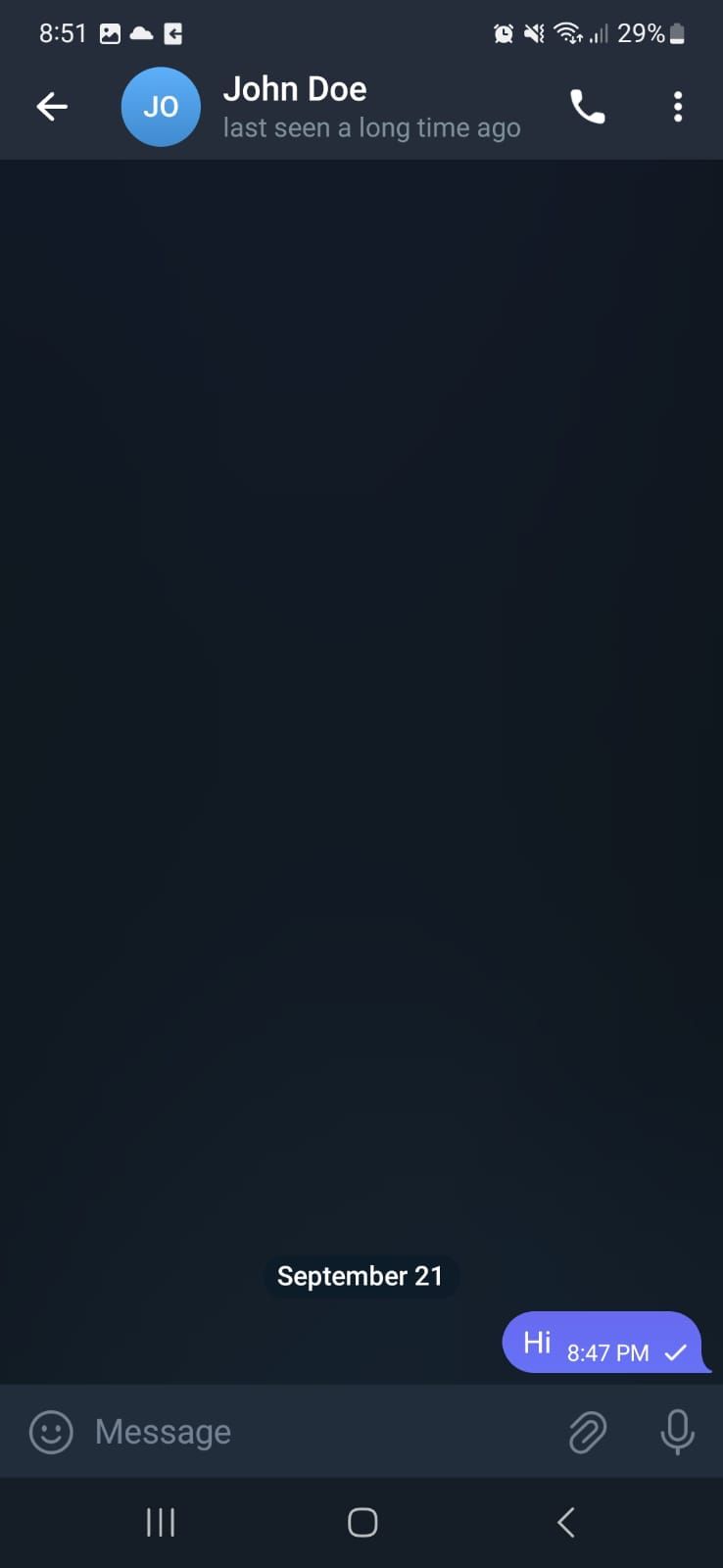This image is a screenshot from an Android phone capturing a conversation. The notification bar at the top displays the time as 8:51 along with various icons including a photo icon, a cloud icon, and a rectangle with a left arrow in the middle on the left side. On the right side, additional icons are visible: an alarm clock, vibration status, WiFi signal strength, 4G signal strength, and a battery indicator showing 29% charge.

Below the notification bar, the contact name "John Doe" is prominently displayed. Beneath the contact's name, it indicates that John Doe was "last seen a long time ago." The screenshot further reveals a single message in the conversation: a text from the user saying "hi" sent at 8:47 on September 21st. The entire screenshot is rectangular in shape, capturing this concise exchange.